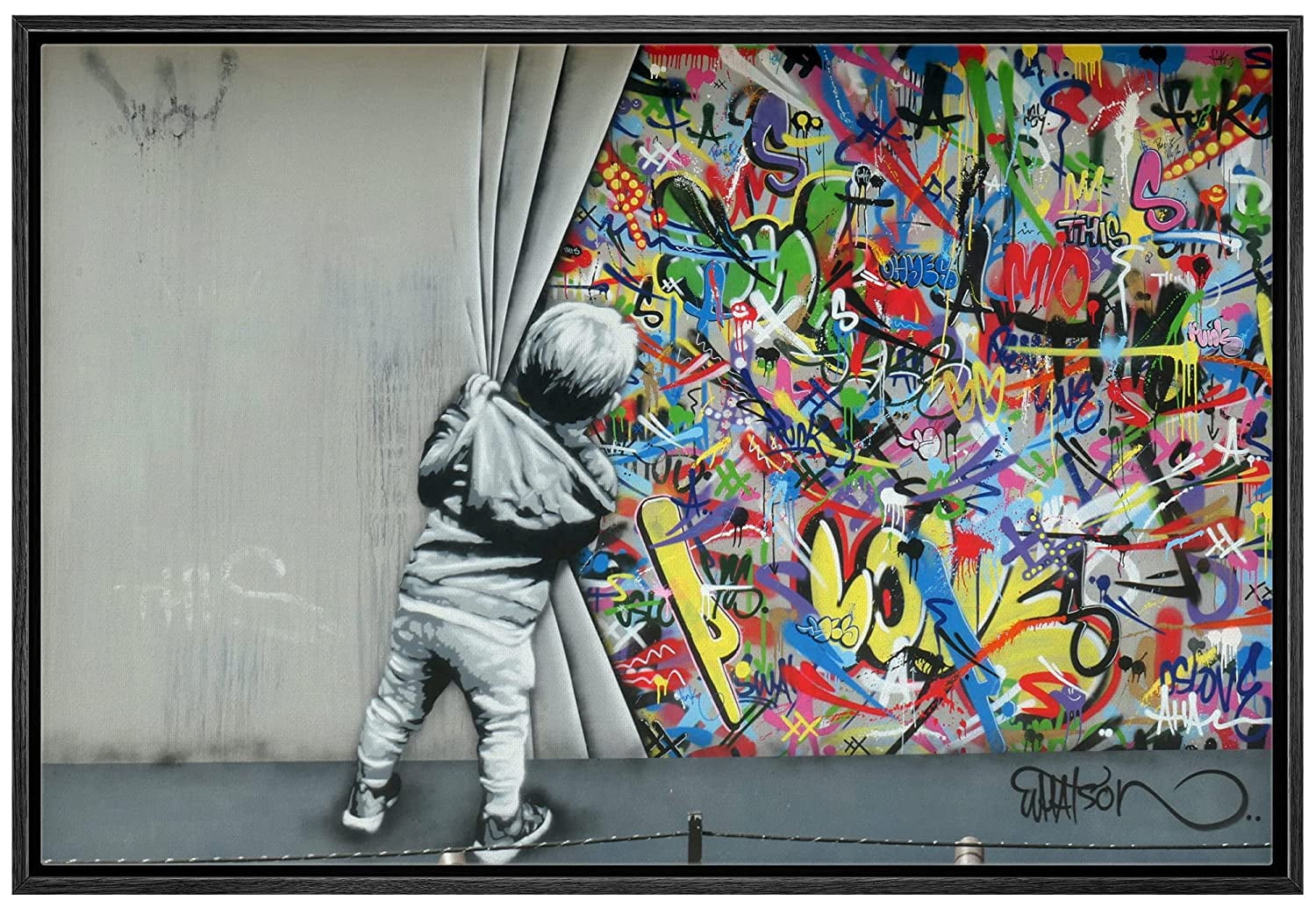The image is a detailed painting capturing a poignant scene where a small child, perhaps two to three years old, is depicted in grayscale, pulling back a gray curtain to unveil a vibrant wall of graffiti. This toddler, dressed in a hoodie, jeans, and tennis shoes, stands on a gray platform while holding the gray curtain, which features the faint word "THIS" and a dim 'W' at the top left. The wall behind the curtain bursts with bright colors, showcasing graffiti in purples, pinks, greens, reds, yellows, and blues. Among the vivid spray-painted letters and words, "LOVE" appears multiple times, and the letter 'S' is repeated throughout. The artwork is signed by the artist at the bottom right, reading "Watson."